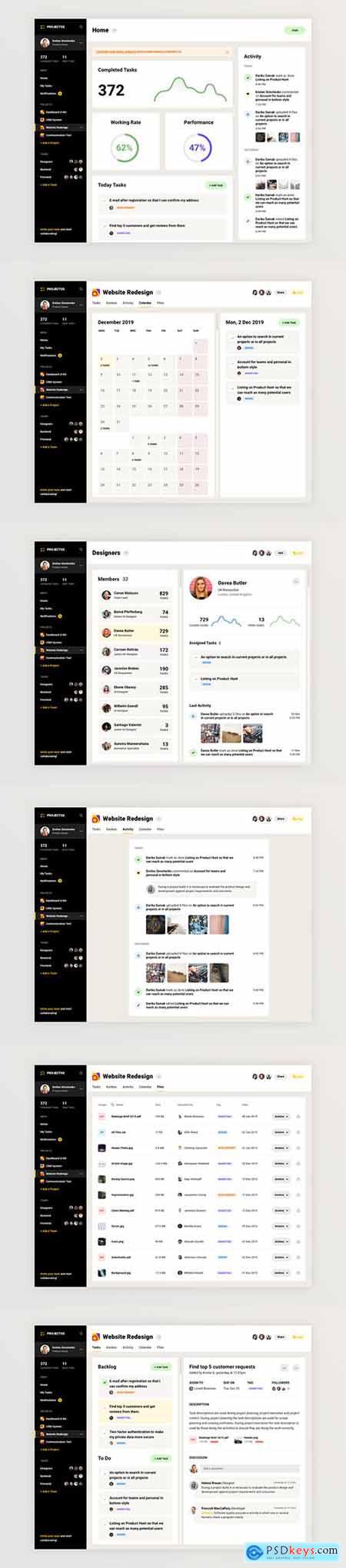This series of images showcases six different screenshots, presumably from a desktop or laptop interface. Here's a detailed breakdown of each:

1. **Screenshot One**:
   - **Left Side**: Features a black vertical bar.
   - **Right Side**: Displays a graph, with detailed observations below:
     - **Underneath the Graph** (towards the right): A half-circle outlined in purple, with the remainder in light gray.
     - **Left of the First Circle**: Another circle, about three-fourths to two-thirds outlined in green, both containing central numerical values (unreadable).
     - **Top Area (Left Side)**: Bold dark gray text displaying "372."
   - **Top Left Header**: An orange banner covering approximately three-fourths of the window's width.
   - **Right Side of the Orange Header**: A large white rectangular area detailing a list view, with numerous small black texts.
   - **Top of the Orange Area (Left Side)**: Black bold header text.

2. **Screenshot Two**:
   - **Calendar View**:
     - **Left and Middle Sections**: Several gray boxes.
     - **Right Side**: Two columns of light red boxes.
   - **Far Right Section**: A thick white rectangular block with a gray bubble, housing three descriptions or status updates in black text.
   - **Left Side Menu**: A vertical menu with a black background.

3. **Screenshot Three**:
   - **Left Side Menu**: Same long black vertical rectangle from the previous screenshots.
   - **Main Area (Right Side)**: Numerous user images arranged vertically in circular frames.
     - **Beside Each Image**: Bold black writing (names), with lighter text above each.
     - **Far Right**: Ranking indicator; the third item is highlighted in pale yellow, indicating it is selected.

This detailed caption provides a thorough description of the elements and layout presented in each screenshot, capturing the nuances and structures observed.